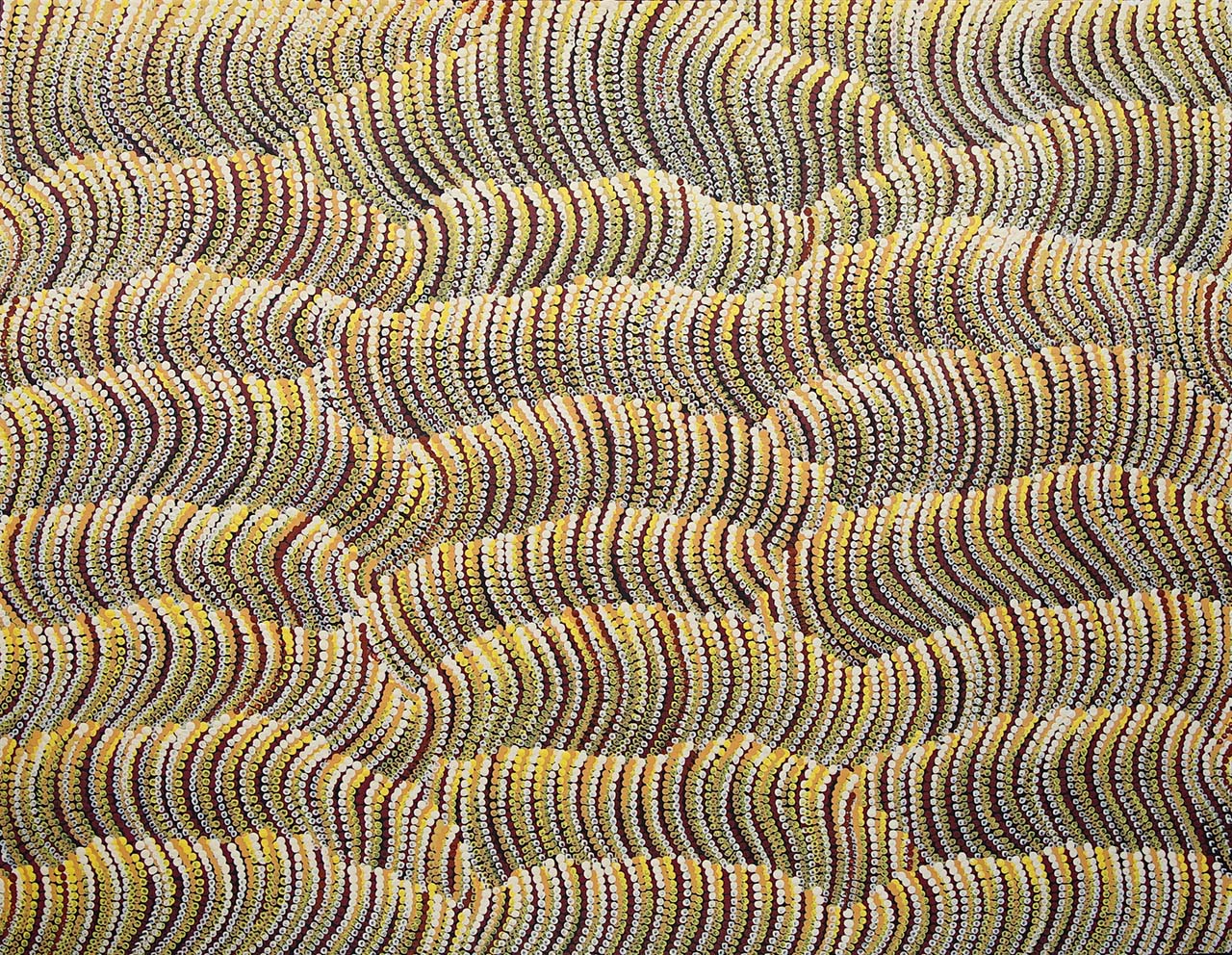The image is a square, multi-colored artwork characterized by rows upon rows of vertical, wavy lines. These squiggly lines create an appearance reminiscent of either caterpillars without distinct legs and faces or hills and waves, covering the entire space without any borders or background. The lines feature a repeated color pattern, predominantly cycling through white, yellow, blue, and occasionally including tan, dark brown, and black. The wavy lines themselves are closely packed creating a mesmerizing, almost cloth-like or bead-like texture. Upon close inspection, some lines seem to form shapes reminiscent of numbers such as zeros, eights, and nines, adding an extra layer of curiosity to the image. Overall, the consistent, undulating patterns of colors and lines make this artwork both intriguing and visually engaging.